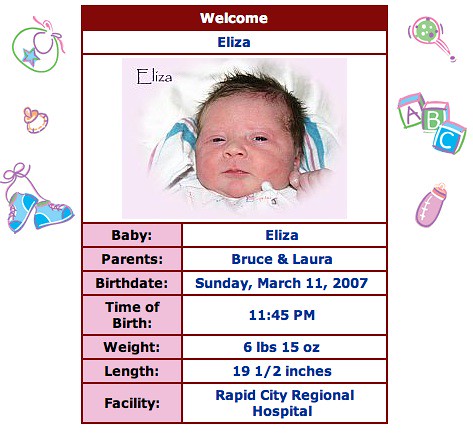The birth announcement for baby Eliza features a welcoming red bar with white text at the top, proclaiming "Welcome." Below this, in a white bar in the upper left corner, is the baby's name, "Eliza," situated above a photo showcasing only the baby's face, set against a blue-patterned blanket. The layout includes two columns of detailed information: on the left, the headers such as "Baby," "Parents," "Birth Date," "Time of Birth," "Weight," "Length," and "Facility" are displayed in black text against a pink background. Correspondingly, on the right, the specific details are provided in blue text: "Eliza," "Bruce and Laura," "Sunday, March 11, 2007," "11:45 p.m.," "6 pounds 15 ounces," "19 1/2 inches," and "Rapid City Regional Hospital." Surrounding this information is a red rectangular border, and adorning the right side of the image are playful graphics of baby items including bibs, baby shoes, pacifiers, rattles, blocks, and bottles, adding a charming touch to this joyous announcement.